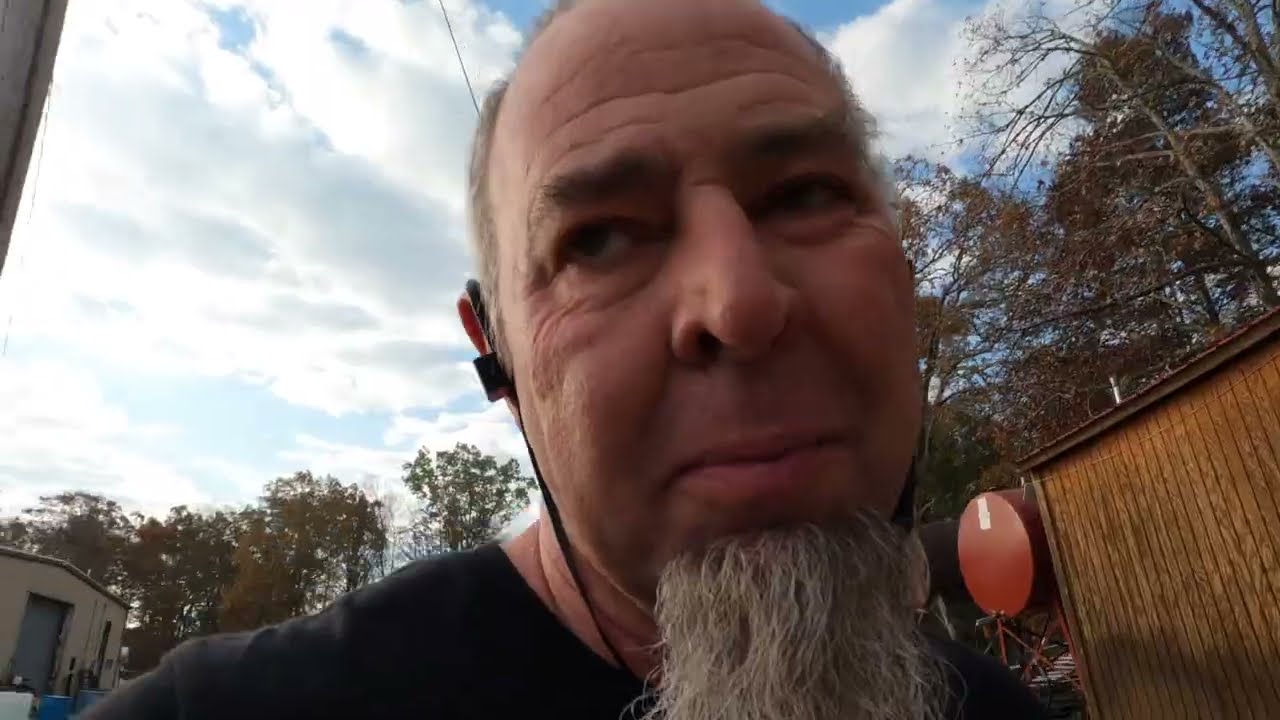Close-up of an elderly man with dark brown eyes, an expressive and slightly forlorn face tilted slightly to the left. He has a long, gray goatee that contrasts with his otherwise clean-shaven face. Black headphones rest over his ears, and he wears a black shirt. His head is set against a backdrop of a diverse natural and built environment.

To the right of the man, a brown wooden shed with a large orange metal tank featuring a white square and a gray outlet is visible. The shed is framed by another light brown building with brown trim and a light gray door, peeking through on the left side of the image. The surroundings feature a mix of tree types: bare branches indicating autumn, evergreen trees, and trees displaying amber foliage. The sky, filled with green and white clouds, allows light to filter through, adding a soft, radiant glow to the image.